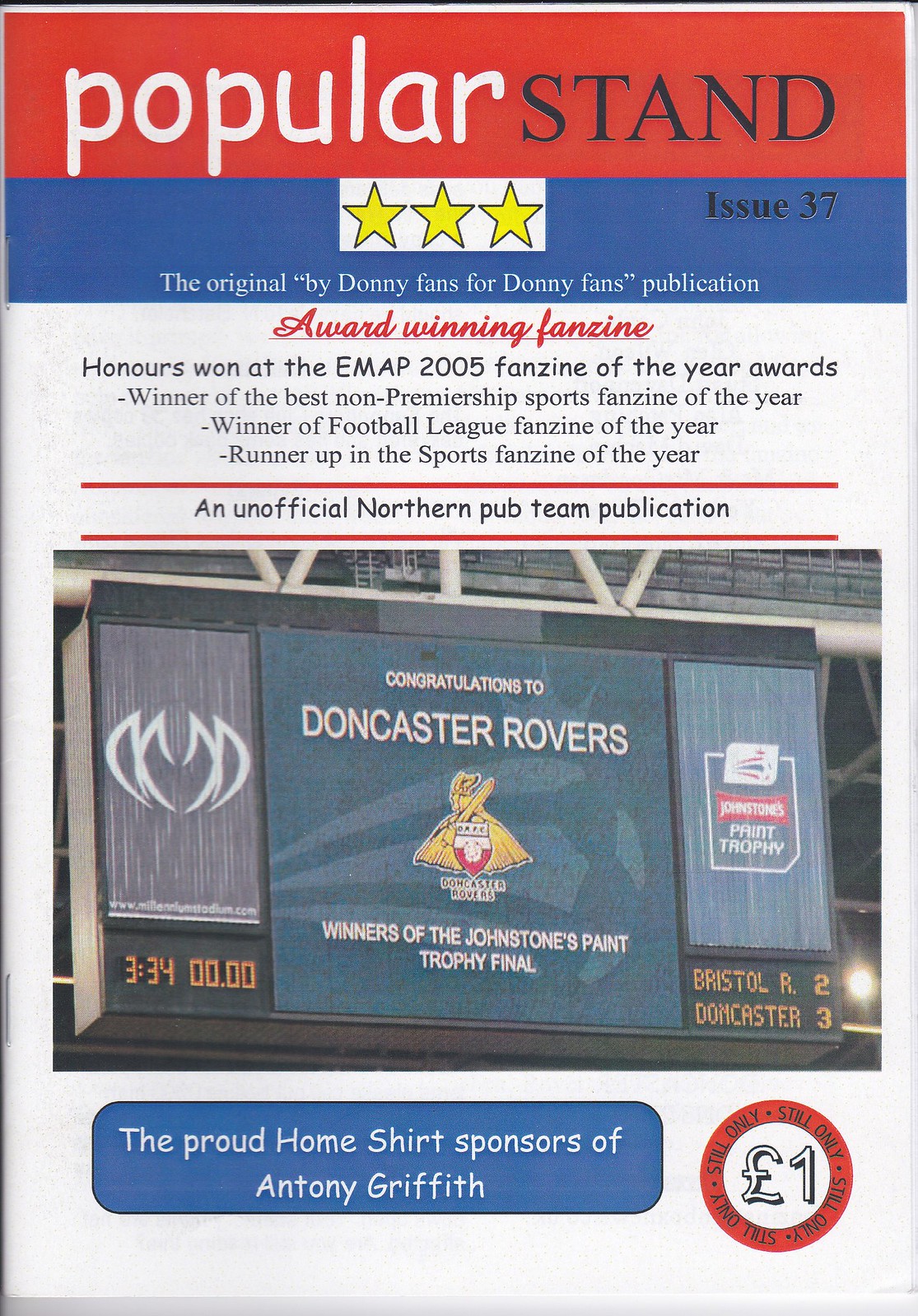The image is a detailed front cover of the magazine "Popular Stand," specifically Issue 37. Dominating the top portion is a red banner with the magazine's title; "Popular" is written in lowercase white letters, and "Stand" in uppercase black letters. Below this, there is a blue horizontal bar with a smaller white inset containing three gold stars, and to its right, "Issue 37" is written in black on the blue background. Centered beneath the banner, in white letters on the blue background, it reads, "The original by Donny fans for Donny fans publication."

The middle section of the cover prominently displays the accolades of the magazine. Written in black text on a white background, it lists: "Award-winning fanzine," followed by various honors such as "Winner of the Best Non-Premiership Sports Fanzine of the Year," "Winner of the Football League Fanzine of the Year," and "Runner-up in the Sports Fanzine of the Year," referencing the EMAP 2005 Fanzine of the Year Awards.

A red line demarcates this text from the next section, which reads, "An unofficial Northern Pub team publication," and then another red line separates this from the lower part of the cover which features an image. The image appears to be a scoreboard display from a Doncaster Rovers match, indicating topics covered in the issue.

On the left side of the scoreboard, gray and light blue sections include a digital clock showing "3:34" and another display reading "00:00". The center of the scoreboard displays a yellow emblem and reads, "Congratulations to Doncaster Rovers," with additional text that mentions their victory in the Johnstone's Paint Trophy Final. On the right side, yellow digital writing records the score Bristol R.2 Doncaster 3.

Below the scoreboard image, a blue rectangular box at the bottom contains white text stating, "The proud home shirt sponsors of Anthony Griffith." Nearby, a bold red circle repetitively states "Still only" around the edge, and in its center is a white circle with the British pound symbol (£) and the number one, highlighting the magazine’s price of £1.

Overall, the cover displays the magazine as a proud, fan-driven, award-winning fanzine associated with Doncaster Rovers.